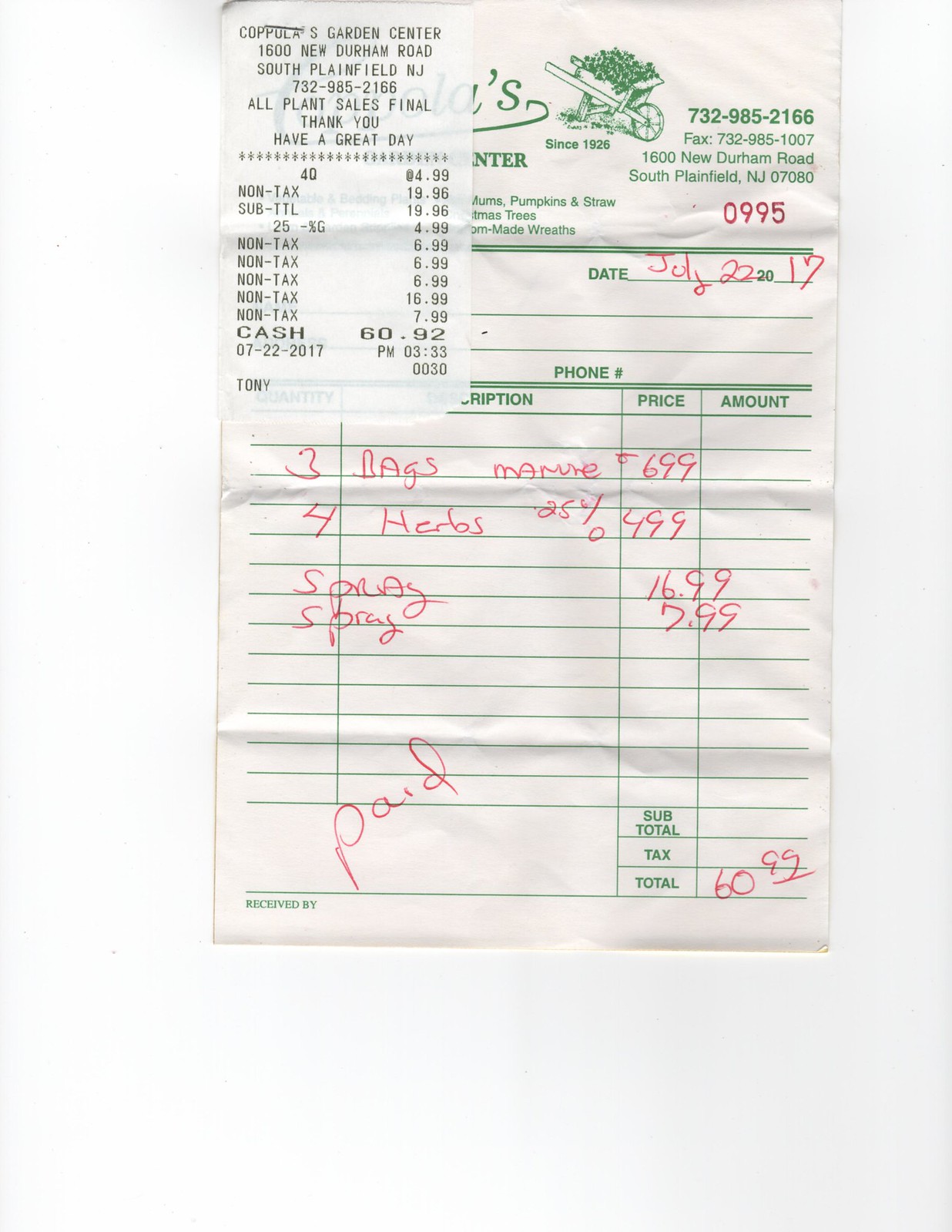This close-up photograph captures a detailed handwritten receipt from Coppola's Garden Center. The white receipt paper prominently features green text, which includes the name, logo of a wheelbarrow filled with plants, phone number, fax number, and address of the garden center, along with a brief description of their offerings. Handwritten in bright red pen are the purchased items: three bags of manure at $6.99 each, four herbs discounted at 25% for $4.99 each, and two types of spray priced at $16.99 and $7.99. The total amount due is listed as $60.99, with "paid" noted in red script at the bottom. Stapled to the top left corner of this handwritten receipt is a smaller printed register receipt that reiterates the total and includes a thank you message and the garden center's address,  New Durham Road, Plainfield, New Jersey. The image background is entirely white, providing no additional context or items.